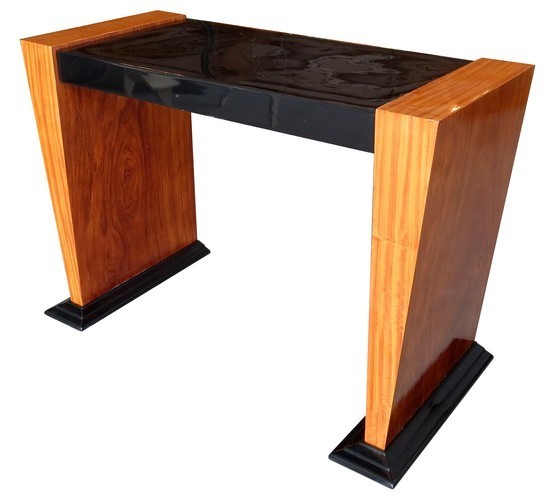The image depicts a minimalist, modern piece of furniture set against a plain white background, featuring a simplistic yet unique design. This structure resembles a desk or a stool and comprises two wide, light wood-colored legs that taper upwards in a reverse triangle shape, a distinctive design choice. The base of these legs is black, providing a contrasting accent. The top surface is a sleek black material, possibly resin or marble, giving it a refined, artistic appearance. Despite its desk-like shape, the piece’s low height and unconventional design elements suggest it may serve multiple purposes, blurring the lines between a stool, a nightstand, and a small table. This artistic construction stands alone in the image, highlighting its solitary, sculptural form.